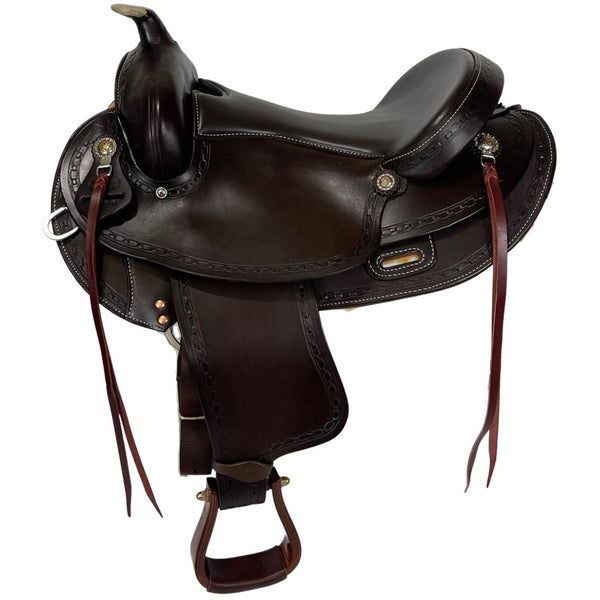The image depicts a meticulously crafted horse saddle, predominantly made of dark brown, almost black, shiny leather. The leather appears soft, smooth, and beautifully finished, suggesting high quality. The saddle is relatively rounded, featuring a horn at the front oriented towards the left from the viewer's perspective. Notably, it includes a backrest area for added rider comfort.

Decorative elements are modest but elegant. There is intricate white stitching around the edges, adding accent without overwhelming the design. The saddle also sports some ornamental work near the fringes where the rider would sit. Additionally, there are a few brass and silver buttons—three silver ones at the top and two smaller gold ones at the bottom—which lend a subtle yet sophisticated sparkle.

Hanging from the saddle are leather tassels or strips in a lighter, warmer brown hue. These tassels attach to silver medallions and extend to about two feet in length, tapering to a point at the end. A red leather strip can also be seen, adding a slight contrast to the overall dark theme. 

Functional components include sturdy stirrups, crafted from the same dark leather, and reinforced with additional brown wraps to provide a secure footing for the rider. The saddle's structure and detailing suggest a blend of comfort, style, and practical utility, making it a fine example of equestrian craftsmanship.